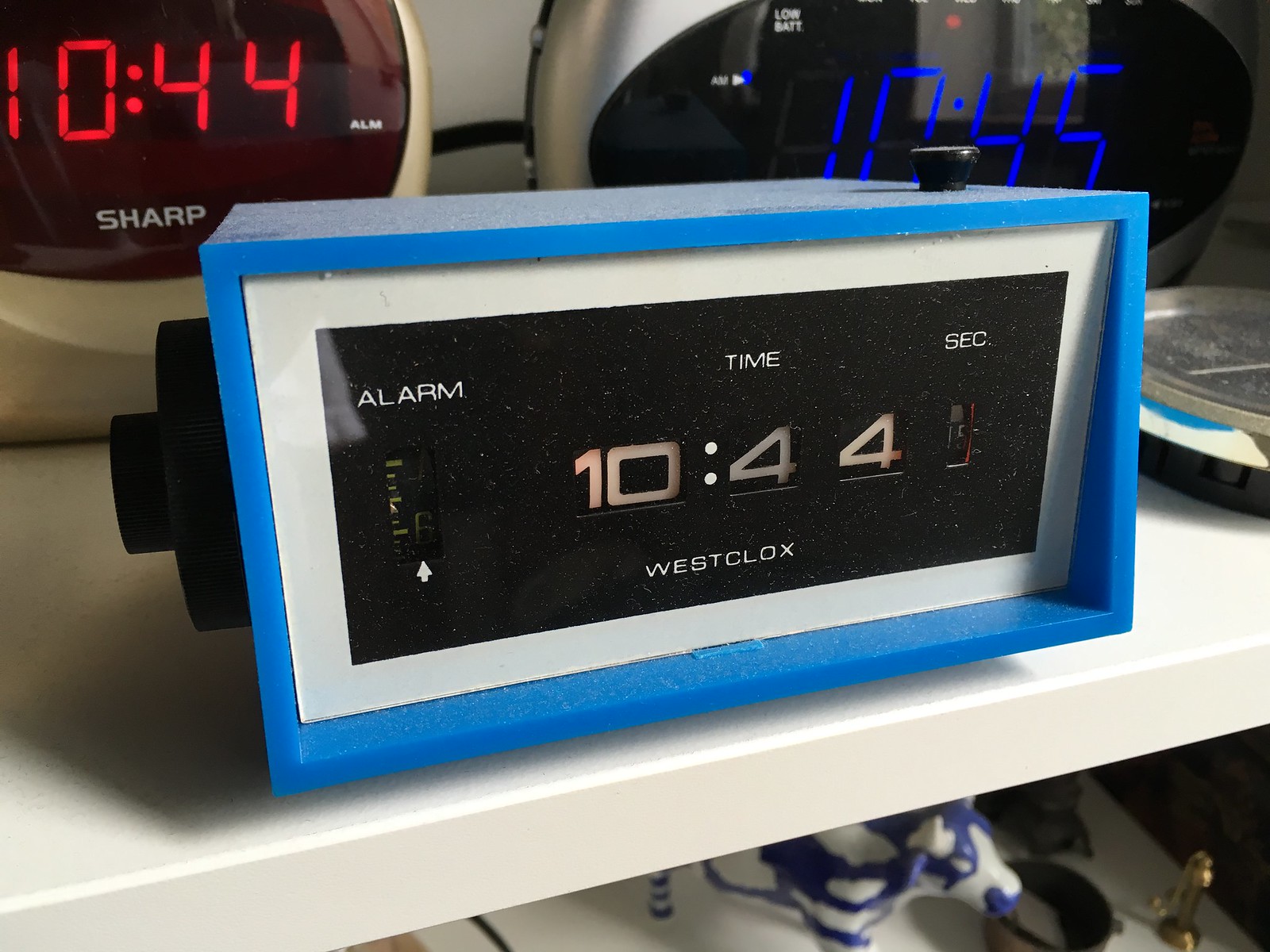This photograph captures three distinct alarm clocks placed on a shelf, each showcasing unique designs and settings. In the foreground stands a Westclox alarm clock, prominently featuring a rectangular blue body with a white border surrounding its black clock face. The time displayed is 10:44. The clock face is detailed with three segments: an alarm indicator on the left, the current time in the center, and seconds on the right. Below the time, the Westclox logo is clearly visible. A small dial beneath the alarm setting, paired with an upward-pointing arrow, offers additional functionality.

Directly behind the Westclox is a more rounded, oval-shaped Sharp alarm clock. This clock is primarily white, with vibrant red numbers displaying the same time of 10:44. "Sharp" is prominently branded on the clock's face, affirming its identity.

To the right, a portion of another oval-shaped alarm clock is visible. This clock features a black face with gray sides, top, and back, slightly obscured but clearly set to 10:45.

All three clocks are neatly arranged on a shelf. Above them, another shelf holds a charming ceramic blue and white cow, adding a whimsical touch to the scene.